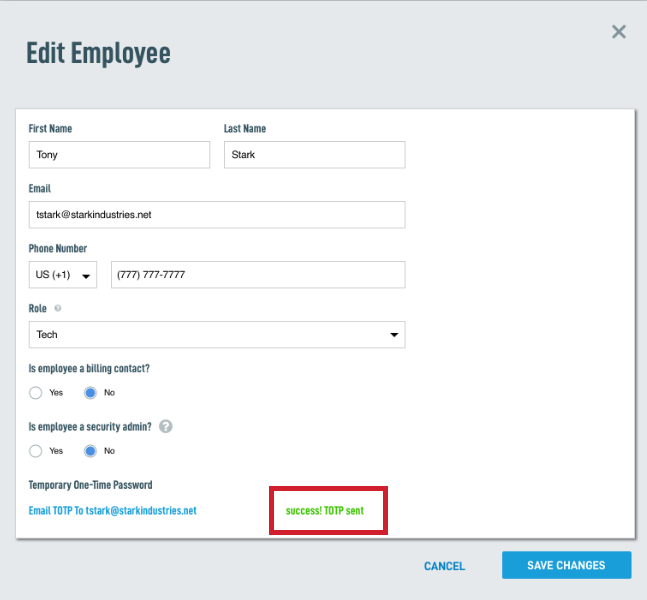The image is a screenshot showing an "Edit Employee" form interface with a gray background overlaid by a white section containing various fields. Starting from the top, the form includes:

1. **First Name:** Filled in with "Tony."
2. **Last Name:** Filled in with "Stark."
3. **Email:** Displayed as "tstark@starkindustries.net."
4. **Phone Number:** Comprising a dropdown menu for the region set to "U.S. (+1)" and the phone number "777-777-7777."
5. **Role:** Selected from a dropdown menu and set to "Tech."
6. **Is Employee a Billing Contact?:** Includes Yes/No buttons, with "No" selected.
7. **Is Employee a Security Admin?:** Again, Yes/No buttons are shown, with "No" selected.
8. **Temporary One-Time Password (TOTP):** Set to be emailed to "tstark@starkindustries.net," with a confirmation message stating "Success: TOTP sent."

At the bottom of the form, there are two actionable buttons: "Cancel" and "Save Changes."